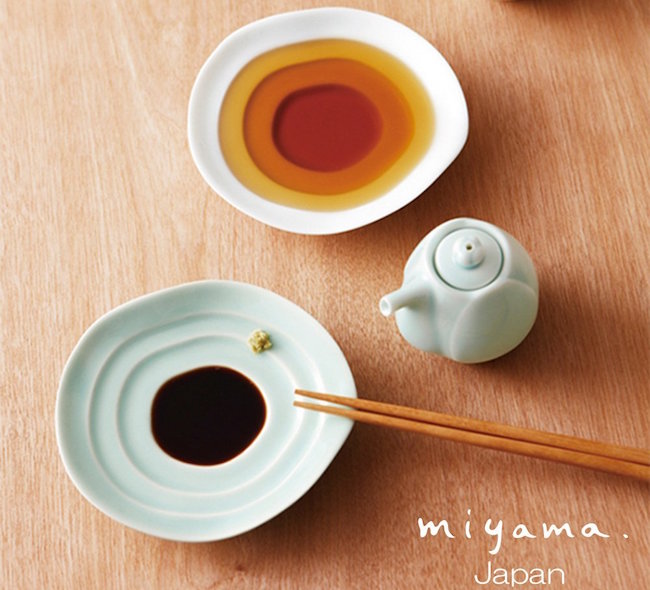The photograph captures an elegantly arranged table setting on a pristine, light wood grain table. The table is adorned with two distinct plates and a miniature teapot. At the top of the image, a unique, almost circular white porcelain dish features three concentric circles of liquid – a red circle in the center, surrounded by an orange ring, and encircled by a yellow outer ring, likely indicating different oils. Below this to the right sits a delicate, very light blue teapot with a round lid and a spout pointing slightly downwards. To the left of the teapot is another white plate, showcasing a dark brown liquid in the center, possibly soy sauce, and decorated with subtle white rings. Propped on this plate are wooden chopsticks, extending downwards to the right. The composition is framed within a square-shaped photo, which in the bottom right corner features the text "Miyama" in an artistic font and "Japan" below it in a standard white font.